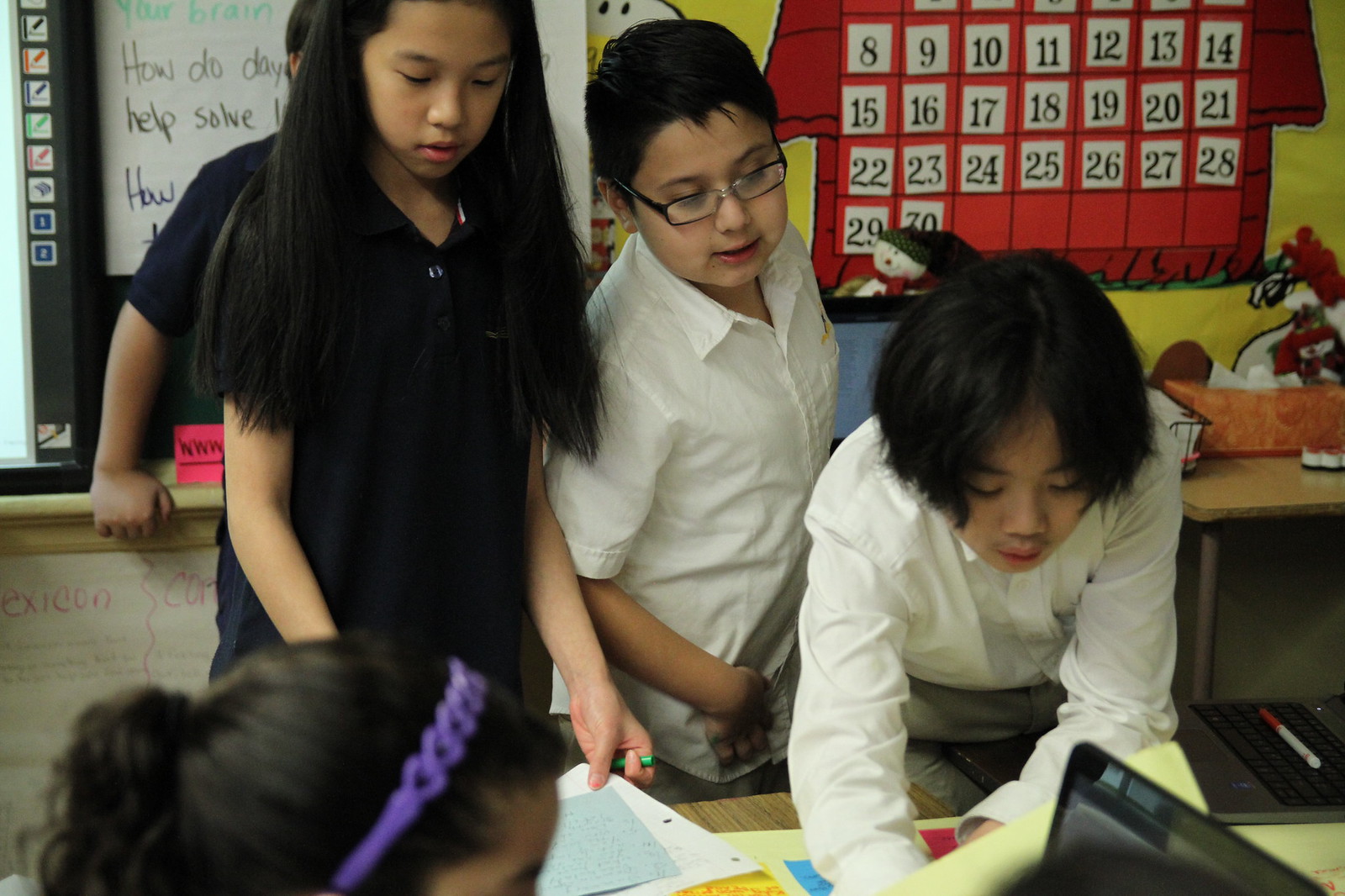In the image, there are four young children, predominantly of Asian descent, gathered in a classroom setting, with a partial view of a girl's head with a purple headband in the foreground. Behind her to the left is a tall girl with chest-length straight black hair, wearing a black shirt, who appears to be concentrating on the table in front of her. Next to her is a boy with short black hair and glasses dressed in a short-sleeved white button-down shirt. On the far right, another boy with nose-length straight black hair is wearing a long-sleeve white button-down shirt and is bent over a table, focused on some papers. Behind the children, a chalkboard features the words "how do they help solve," and to the right of the chalkboard is a red doghouse decoration resembling Snoopy's, which has a calendar with white squares and black numbers. The classroom has an academic atmosphere, with the children appearing engaged in their activities.